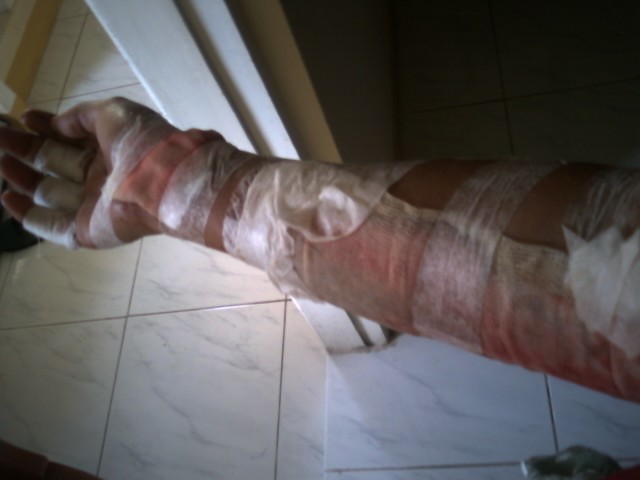In this color photograph, we see a person's extensively bandaged right arm, outstretched and palm up. The arm, visible from just above the elbow to the tips of the fingers, suggests a grievous injury, likely a burn, as indicated by the extensive wrapping and partially translucent bandages. Multiple layers of self-adhesive gauze, some soaked with blood or exudate, cover the arm, with a notably large gauze pad secured at the elbow. Additional pads are meticulously taped on the wrist and upper palm, hinting at severe damage. The setting appears to be a dimly lit hospital bathroom, characterized by a light-colored tile floor with gray marble patterns and a sturdy white doorframe. The image conveys a poignant scene of pain and vulnerability.